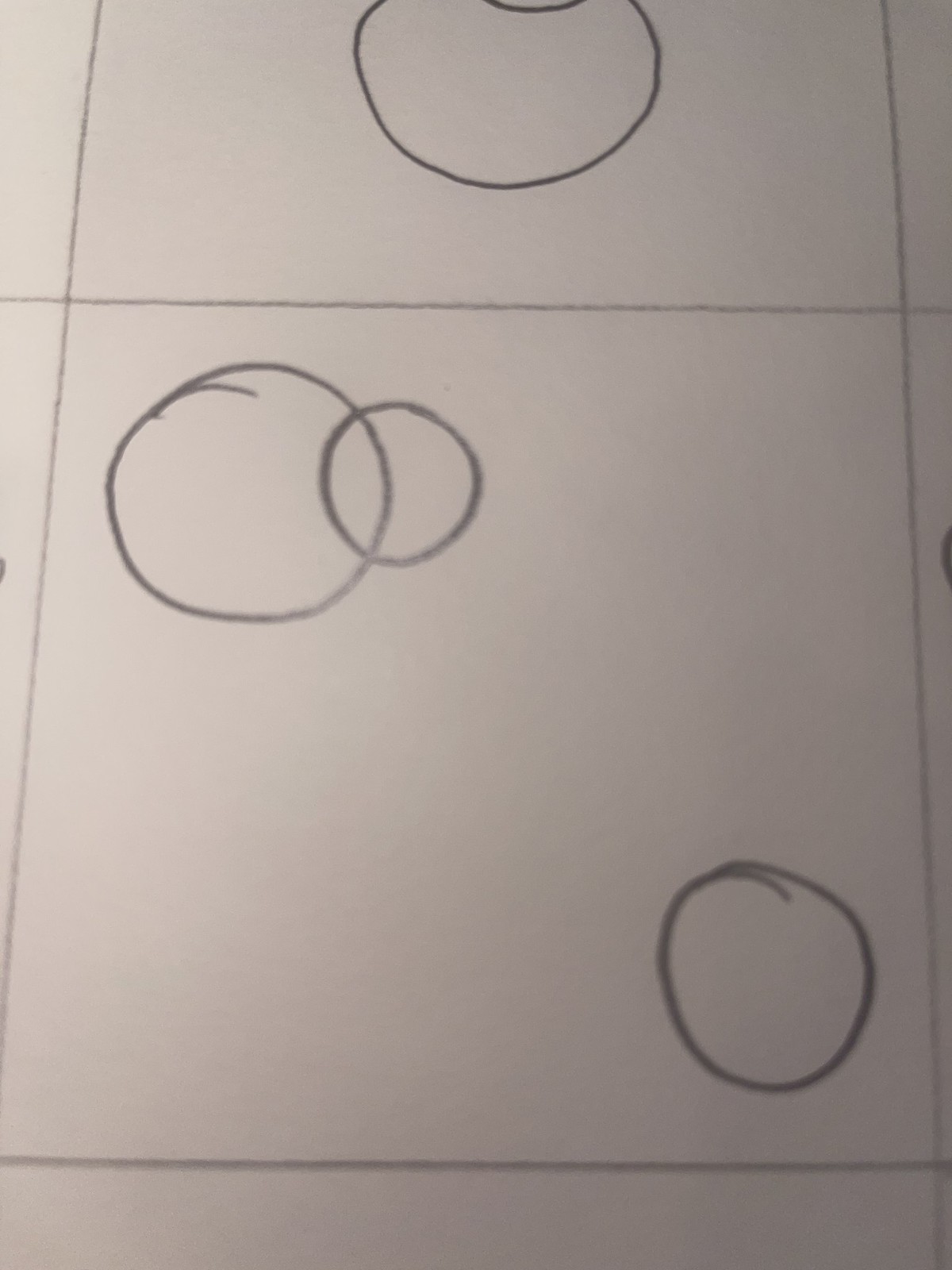A meticulously crafted pencil drawing on off-white paper captures an array of geometric shapes with striking precision. Dominating the composition are two horizontal lines, one positioned near the bottom and another closer to the top, creating a structured layout. From the left edge, another pair of straight lines angles upward, subtly shifting as they follow the right border, forming a grid of squares across the image.

Near the top, within the lower boundary of one of these squares, a partially visible darkened circle emerges, its form truncated by the square's edge. Above, just descending from the top margin, a segment of another circle peeks into view, also rendered in a deeper shade, adding contrast to the composition.

In the square directly below, a trio of circles is carefully positioned. One is situated in the bottom right corner, while another occupies the top left, accompanied by a smaller, overlapping circle. These circles, like the others, are shaded more deeply than the grid lines, drawing the viewer's attention to their placement and contributing to the intricate detail of the artwork.